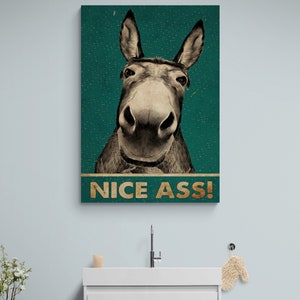The image depicts a humorous scene featuring a prominently displayed painting of a donkey’s face, set against a blue-green background with scattered gold spots. The donkey, which is gray in color with black-tipped ears and beady eyes, is zoomed in and looking directly at the viewer, creating a comical effect. Below the donkey’s face, the text "NICE ASS" is written in all caps in golden letters, adding to the humorous tone. This painting is mounted on a white wall, and beneath it, there is a white structure, possibly a cabinet or a bathroom fixture, with a metallic, L-shaped mechanism sticking up. On this structure, there is a single beige glove hanging on the wall, a lit candle, and a small sprig of flowers in the lower left corner, suggesting a whimsical or decorated setting. The overall scene hints that this could be placed in a public restroom, perhaps in a restaurant or bar, and is intended to amuse viewers with its playful and cheeky message.